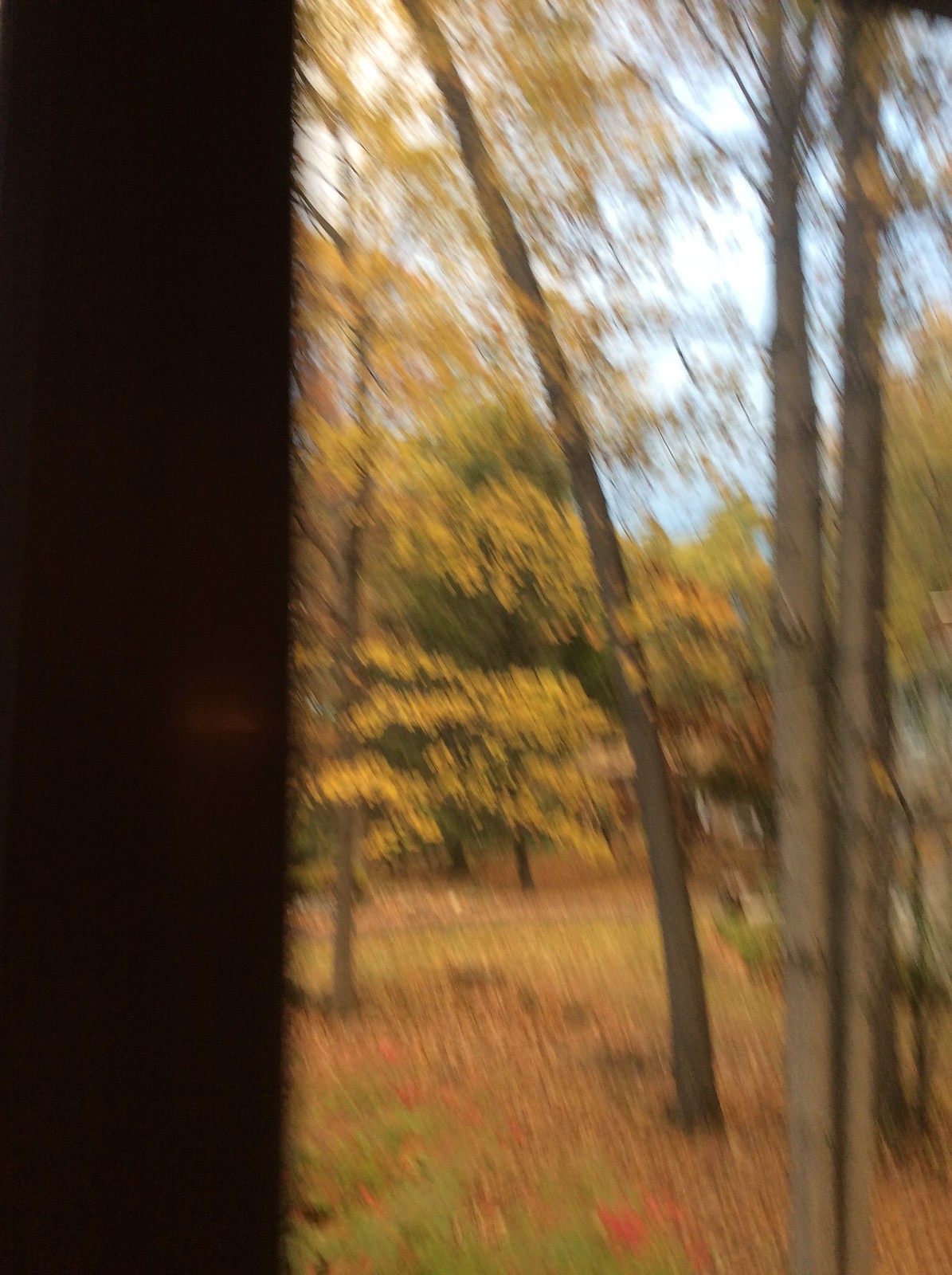In this image, we observe a picturesque outdoor scene, likely captured during the early stages of fall as suggested by the changing leaf colors. The trees scattered throughout the area display a vibrant mix of yellowish-orange foliage with some sporadic green, indicating the transition from summer to autumn. The ground is covered with orange-tinted grass, further enhancing the fall atmosphere.

The left side of the image is obstructed by a dark brown element, potentially part of a structure or some urban feature, giving the scene an intriguing, partially obscured perspective. The photo is illuminated by bright sunlight, casting a warm glow across the landscape and emphasizing the vivid colors of the leaves.

However, the image is slightly blurry, as if taken in haste or with a shaky hand, which makes it challenging to discern finer details. Despite this, the core elements remain visible: the grassy terrain, the cluster of trees adorned with colorful leaves, and the partial obstruction on the left, all under a clear, sunlit sky.